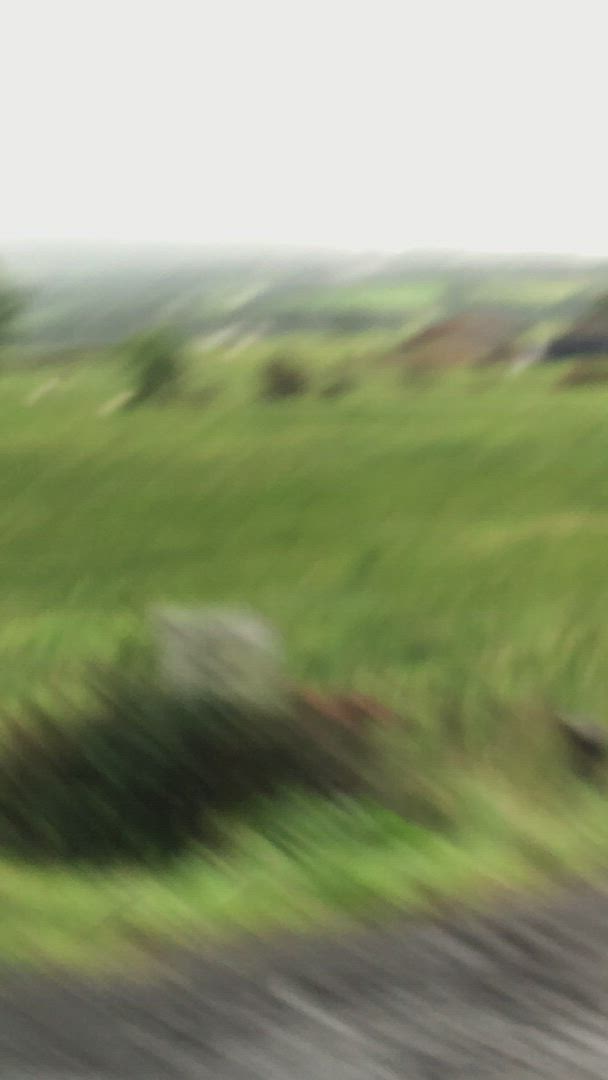In this blurry image, you find yourself standing atop a rugged, dark rocky formation, possibly a pathway or a natural outcrop. Directly before you, nestled among the rocks, lies what appears to be a stone marker, partially enveloped by wild vegetation. The scene then unfolds into vast, undulating grasslands painted in various shades of green. Scattered across these plains are small bushes and, off to the right, a distant brown structure, potentially a house or a church, adds an intriguing element to the landscape. The sky beyond is overwhelmingly bright, almost white, casting a surreal glow over the entire setting.